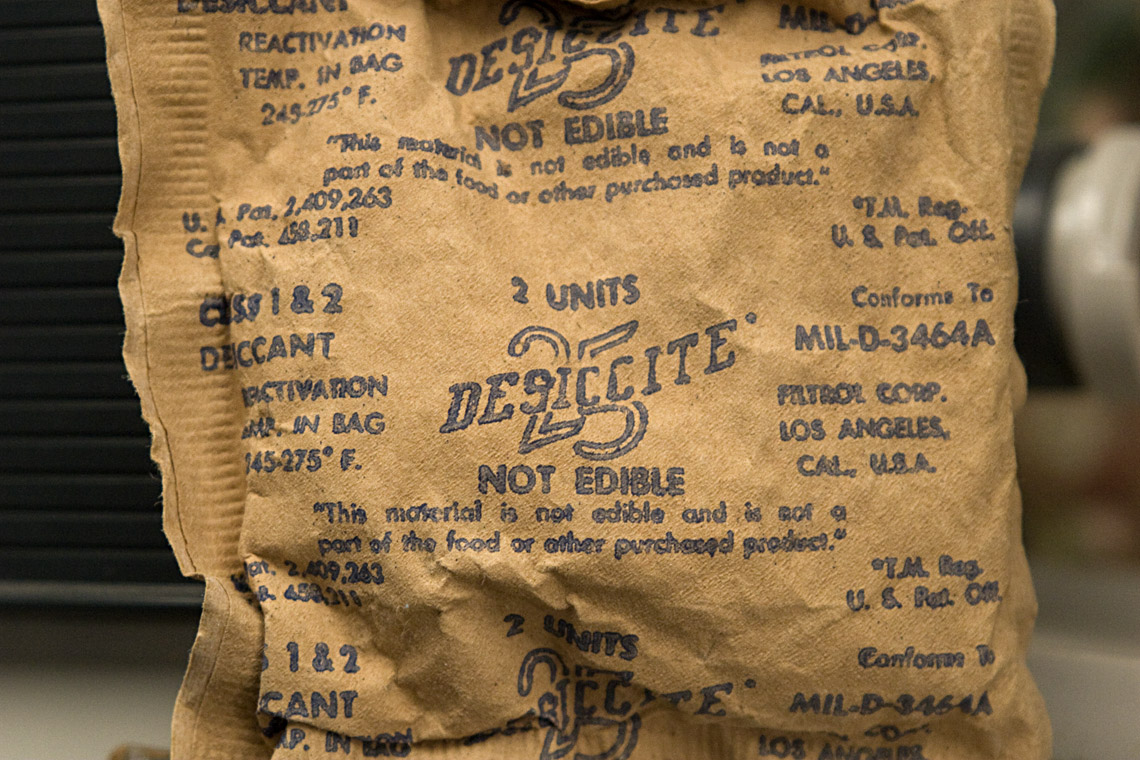In this photograph, a square, brown paper bag is placed centrally on a tan-colored countertop or table, with a dark wall featuring horizontal slats as the backdrop. The bag occupies most of the image, with black text printed across its surface. Prominently, in the center of the bag, the text reads, "Two Units Desiccate," with the word "desiccate" spelled out as "d-e-s-i-c-c-i-t-e." Below this, it explicitly states, "Two Units Not Edible." In parentheses, it clarifies, "This material is not edible and is not a part of the food or other purchased product." Additional text includes the abbreviations "U.S." and "T.M. Bag," and the numbers "1" and "2" can be seen in the lower left corner of the bag. The composition focuses on the bag against the contrasting background, highlighting the details of the text and the material of the bag itself.